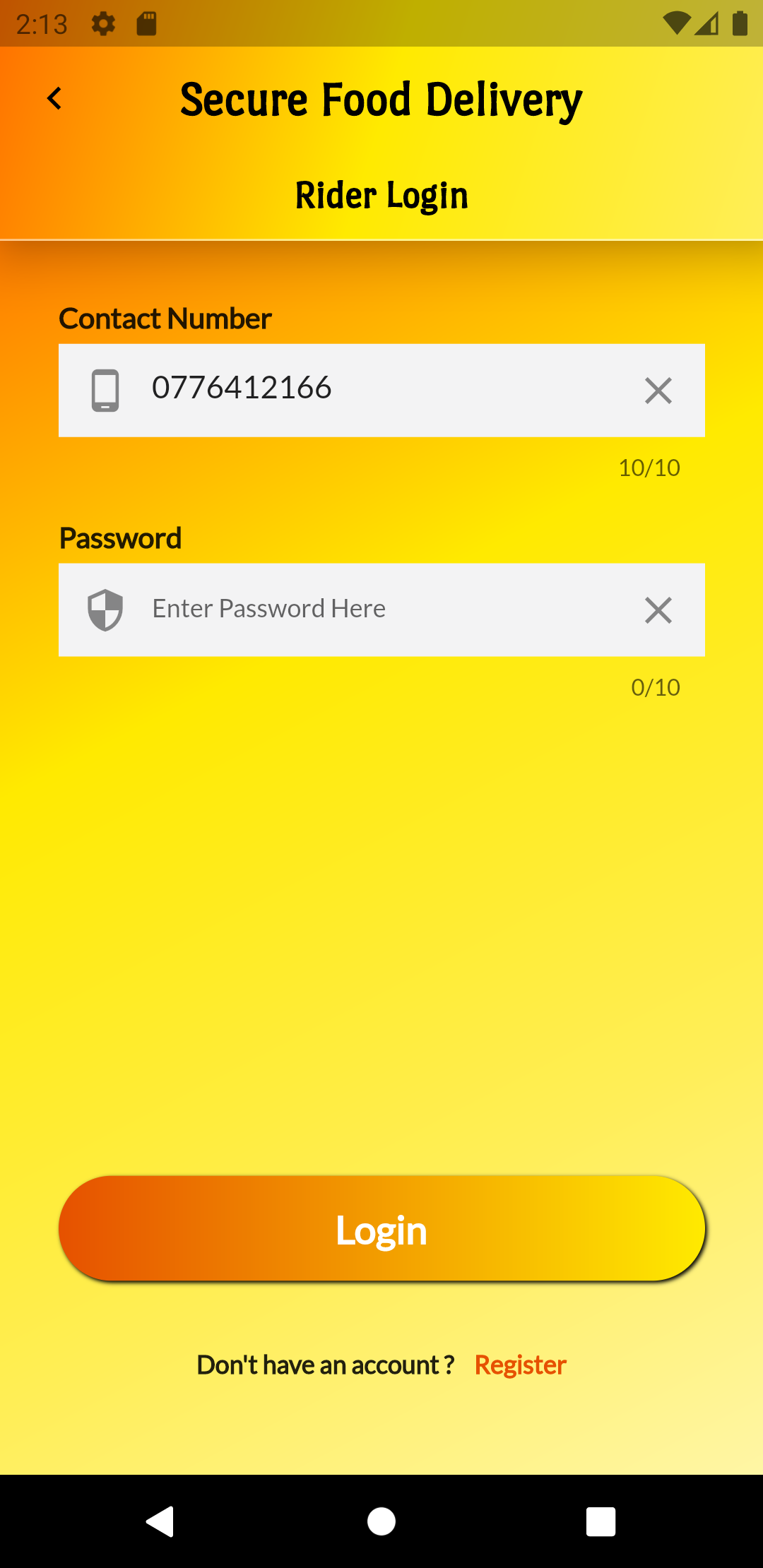In this image, we see a screenshot featuring a vibrant gradient background that transitions smoothly from a warm yellow at the bottom to a soothing orange towards the top, and then back to a mix of yellow and orange at the topmost portion. In the upper-left corner of the screen, there is the number "213" next to a settings icon. On the upper-right side, there are icons indicating that the internet is on and the battery is fully charged. 

Centered prominently on the screen, bold black text reads "Secure Food Delivery," accompanied by an arrow pointing to the left, and the words "Rider Login."

Below this, there are two data entry fields. The first field is designated for the contact number, with instructions in black text above it that reads, "Contact Number." The placeholder in the field displays "07764121661010". Directly below, another section prompts for the password with the text "Password" above an input box that reads "Enter password here." Adjacent to this password field, in the lower right corner, is the text "0/10" indicating the character limit status.